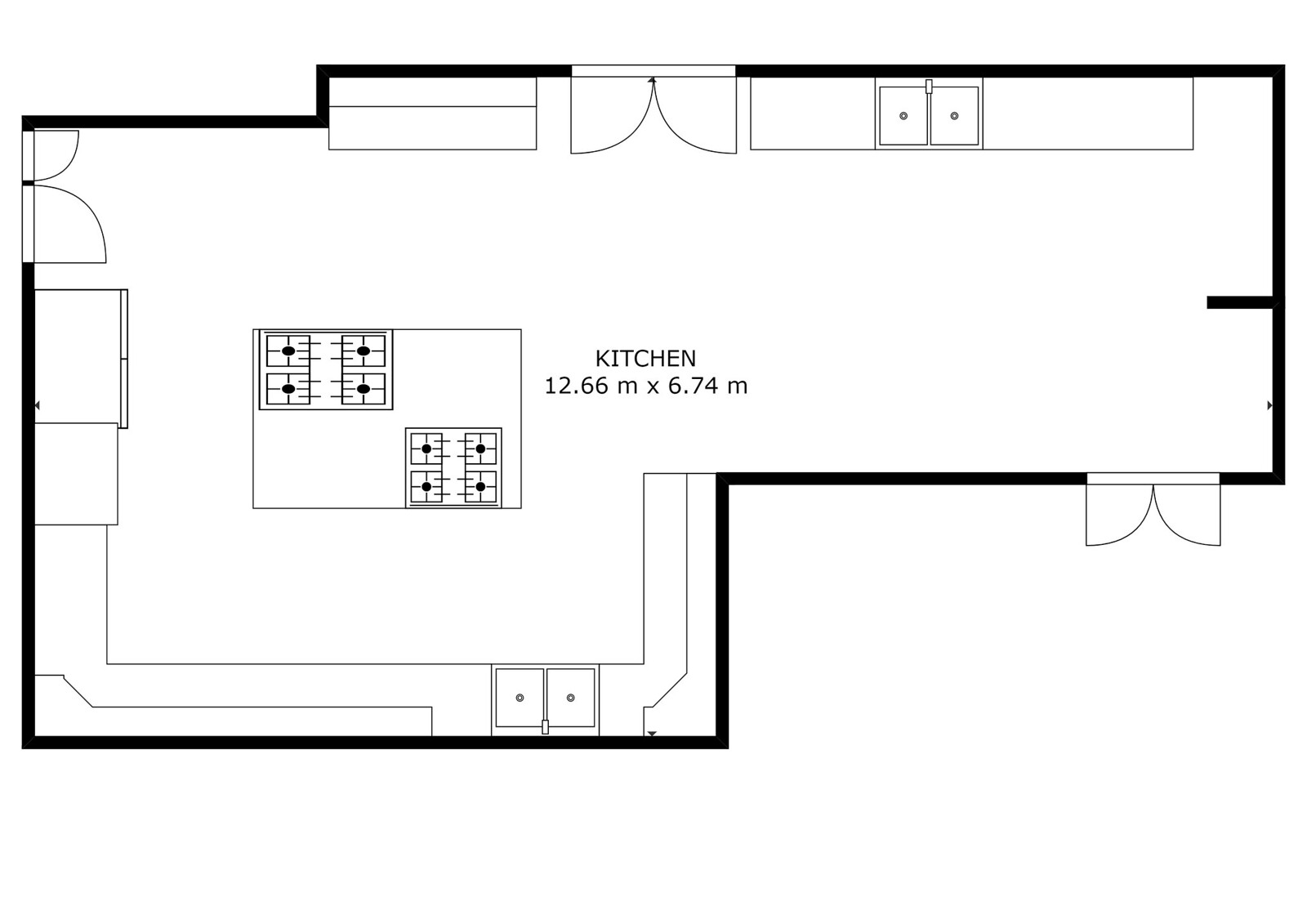This detailed floor plan of a spacious kitchen reveals a square layout with an adjoining rectangular section, confirming its ample size of 12.66 meters by 6.74 meters. At the bottom of the diagram, a continuous stretch of countertops is visible, featuring a centrally located sink. Dominating the middle area is a substantial island equipped with two gas stoves, each boasting four burners, offering extensive cooking capabilities. 

A door symbol is present, indicating an entryway, while the top portion illustrates a series of cabinetry flanking another doorway. Adjacent to this door, an expansive counter with an additional sink is noted, suggesting a dedicated area for food preparation or cleanup. Directly across from this counter, a third door is marked, facilitating multiple access points throughout the kitchen.

Notably, while specific dimensions for the island and other features are not provided, the countertops extend extensively across the kitchen space. The right side of the floor plan, which includes a second sink, appears designed to accommodate a dining table, hinting that this area might serve as a combined kitchen and dining room. With three doors providing varied ingress and egress options, and the potential dining space incorporated, this kitchen is evidently designed to support both culinary activities and social gatherings in a generously proportioned environment.